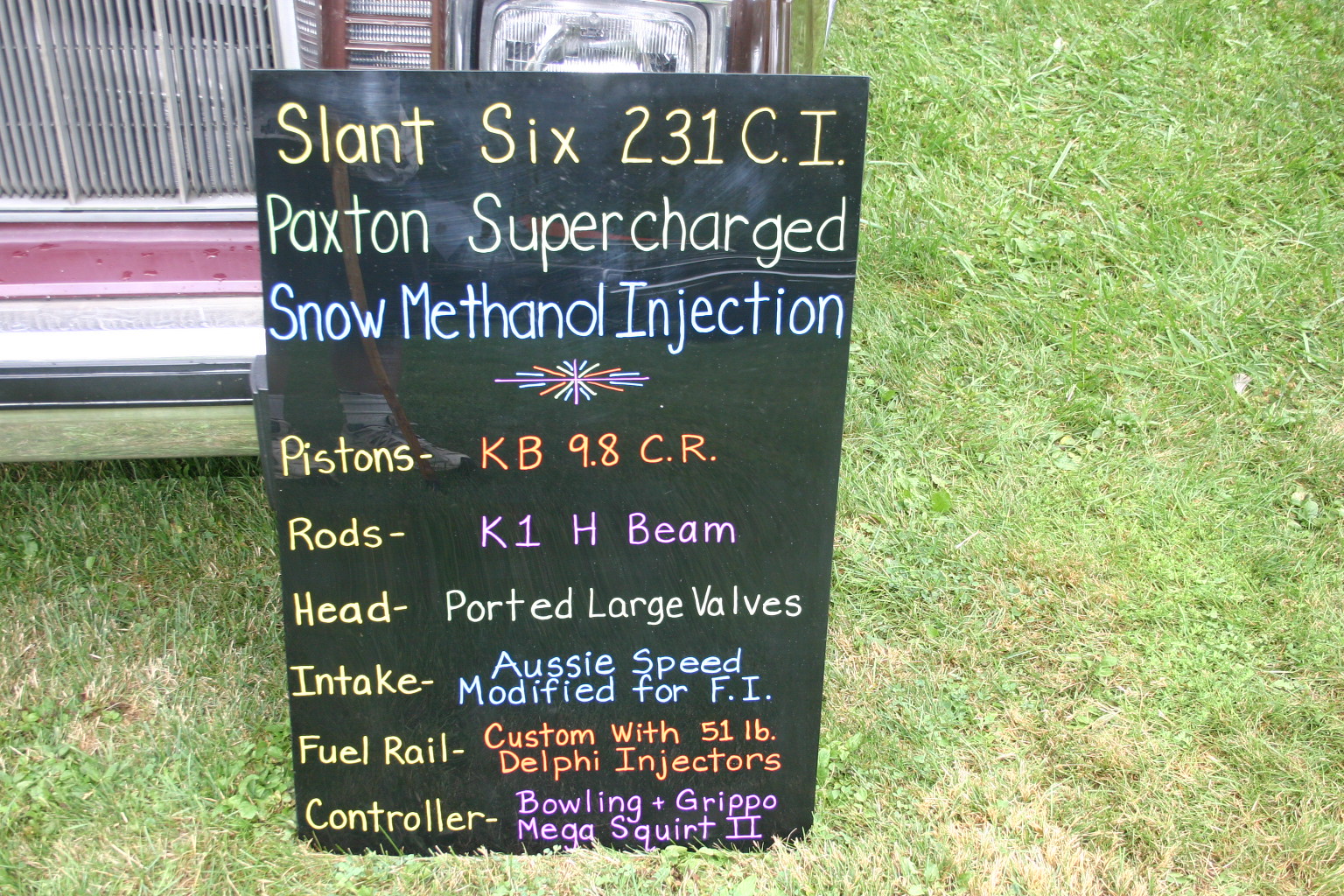This is a detailed outdoor image of a black poster board featuring a comprehensive list of high-performance engine components, which is leaning against the front of a burgundy vehicle parked on green grass. The handwritten sign boasts intricate, color-coded text that reads: "Slant 6231CI, Paxton Supercharge, Snow Methanol Injection, Pistons, KB98.CR, Rods, K1H Beam, Head, Ported Large Valves, Intake, RC Speed Modified for FI, Fuel Rail, Custom with 51lb Delphi Injectors, Controller, Bowling Grip, Megasquirt II." Key terms like "Pistons," "Rods," "Head," "Intake," "Fuel Rail," and "Controller" are highlighted in yellow, while specific details such as "KB98.CR" and "Custom" are in orange, "K1" and "Bowling" in purple, "Ported" in yellow, and "RC" in blue. The sign, reflective enough to faintly show the person taking the photograph, serves as a catalog of modifications for what appears to be a souped-up engine installed in the adjacent car.